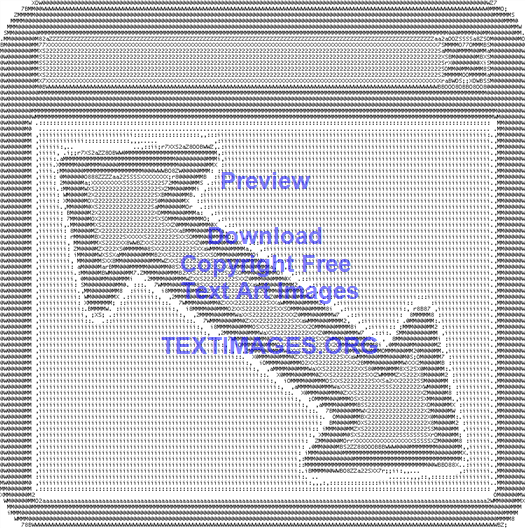The image features a square shape with rounded corners, outlined by a pattern of small black and white dots. The square has a gray border with a lighter gray center, filled with lines or dotted patterns. An X is visible in the upper right part of the square. Central to the composition are two large double-headed arrows, one pointing northwest and the other pointing southeast, characterized by thick, gray sides with black edges. Strategically typed letters form the intricate details. In blue or purple text at the center reads "Preview Download Copyright Free Text Art Images," followed by "textimages.org" in all capital letters below. The overall appearance suggests a meticulously crafted, computer-generated design.